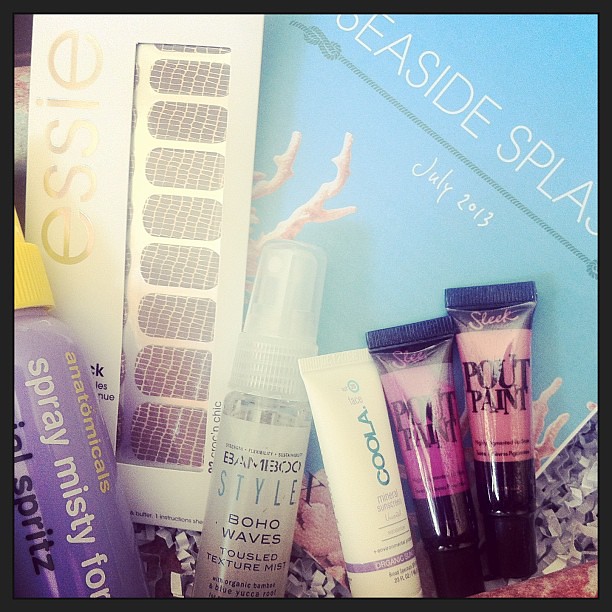The photograph captures an overhead view of a variety of beauty products against a blue background with a black border. At the top left, a white rectangular package with "Essie" written in gold lowercase letters holds what appear to be nail products. Adjacent to it is a purple spray bottle with a yellow lid labeled "Anatomicals Spray Misty for Me Facial Spritz". The largest text on the bottle is "Anatomicals" in yellow, followed by the smaller text "Spray Misty for Me Facial Spritz". Centrally placed is a clear bottle labeled "Bamboo Style Boho Waves Tousled Texture Mist with Organic Bamboo and Blue Yucca Root". There is a white tube marked "KULA Mineral Sunscreen Organic SPF 30" featuring a purple stripe near the bottom. Along the bottom of the image, at the left, are two tubes of Sleek's Pout Paint; the left tube is magenta, and the right tube is a rose color, both with black caps. In the background, a large white card says "Seaside Splash" in white letters against a blue backdrop, with "July 2013" and an illustration of a rope and coral below the text.